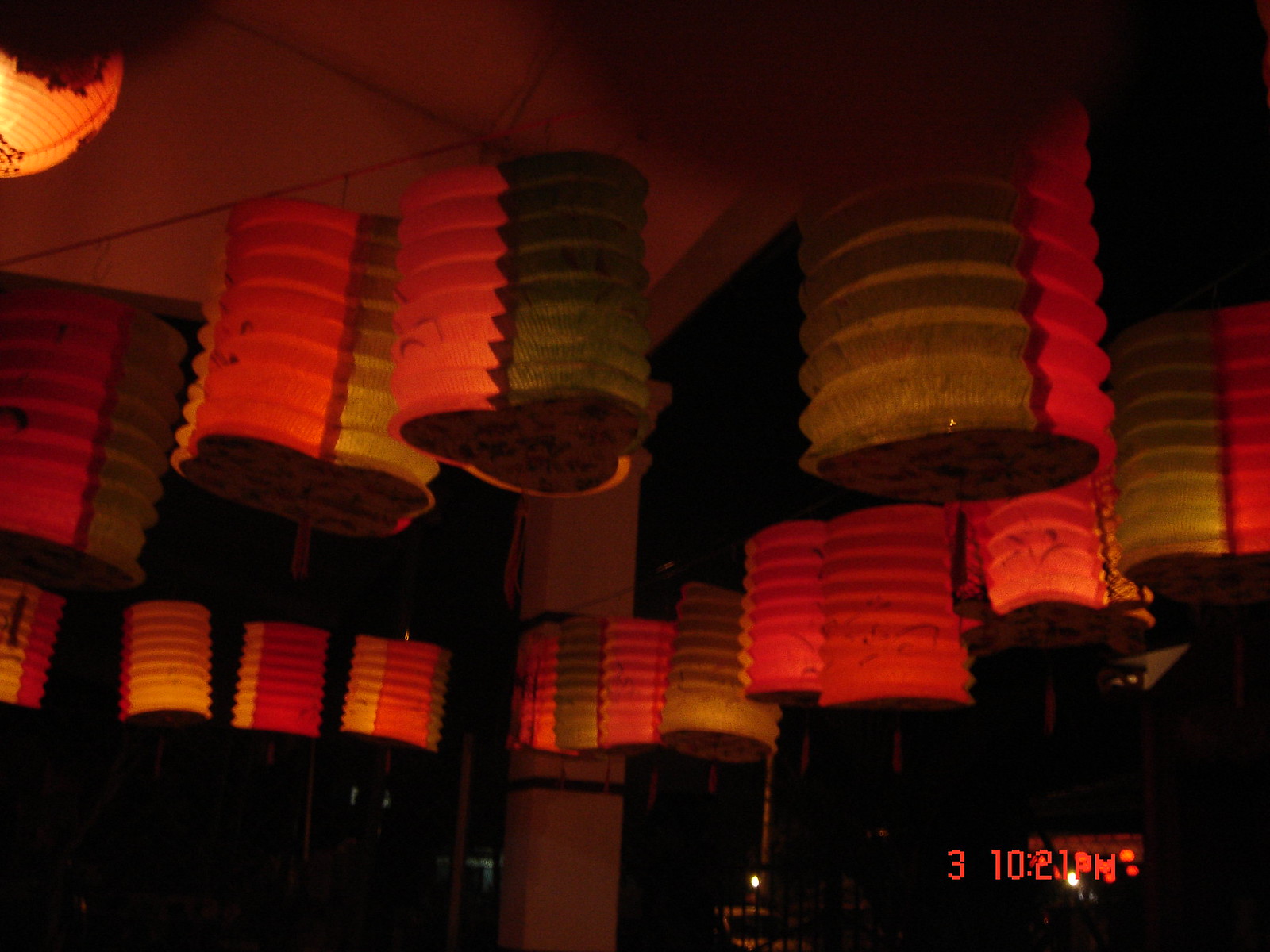The photograph appears to have been taken outdoors, possibly at a restaurant or in an outdoor pagoda-style setting. It features a patio area adorned with numerous Chinese lanterns hanging from a tall ceiling supported by columns. The lanterns, numbering between 15 to 20, vary in colors and patterns, predominantly featuring color combinations like green and pink, orange and green, as well as yellow and orange. These lanterns are accordion-shaped and approximately a foot and a half in length. The scene is set at nighttime, indicated by the glowing lanterns that light up the dark surroundings. Additionally, a digital timestamp reading "3:10 21 p.m." is visible at the bottom right corner of the photograph, despite the clear night sky. The overall ambiance created by the lanterns and the setting is intriguing and visually captivating.